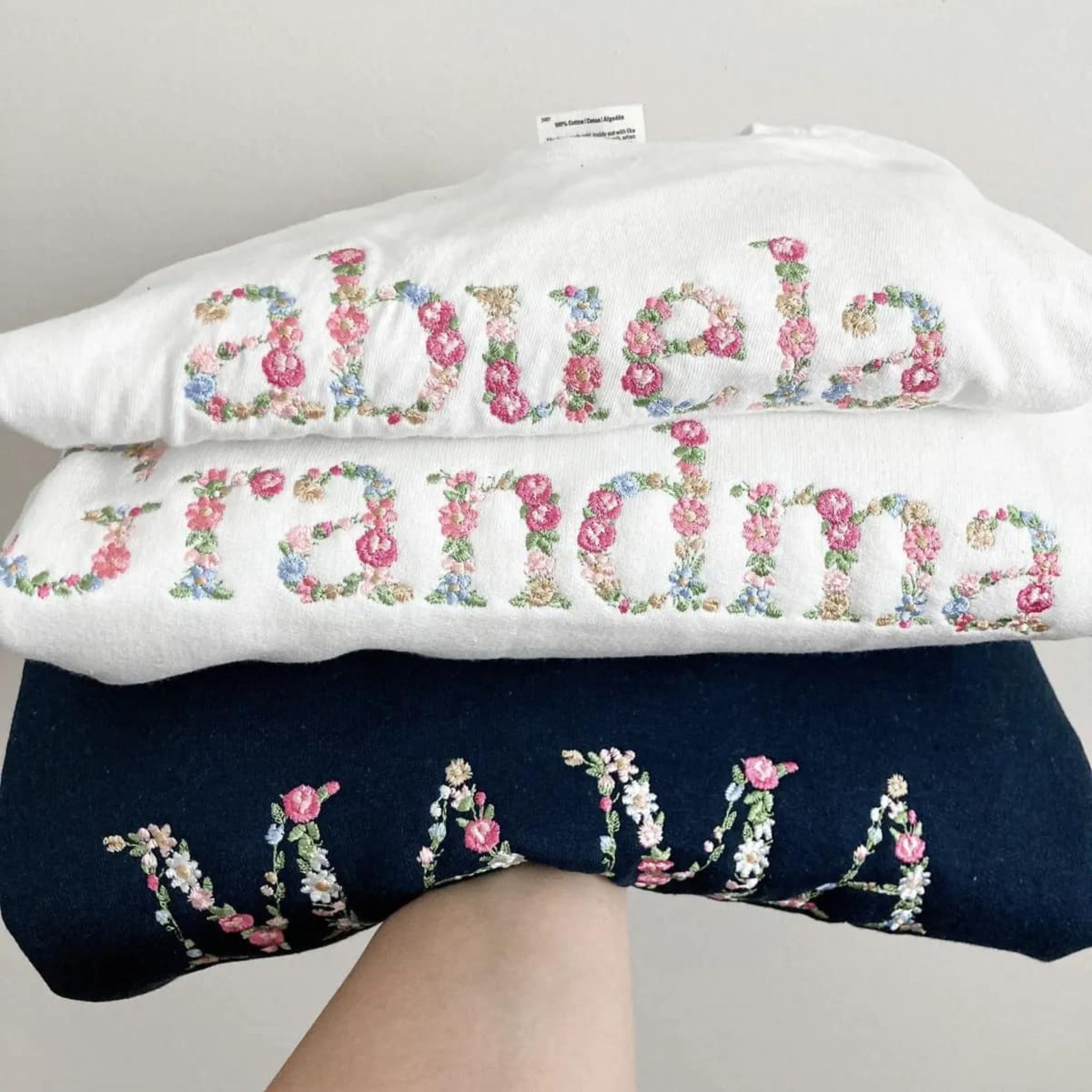The image, set against a white background, appears to be an advertisement photograph featuring an extended, smooth forearm holding a neatly folded stack of three sweatshirts. The sweatshirts are intricately embroidered with colorful flowers forming the letters that spell out familial titles. The top two sweatshirts are white, with the one on top embroidered with "Abuela" and the one beneath it displaying "Grandma." Each letter in these words is intricately crafted from flowers in various shades of pink, blue, white, and green, with elements like buds and leaves adding detail. The bottom sweatshirt is navy blue and features the word "Mama" similarly spelled out with flowers, using a mix of colorful floral designs. The vibrant and detailed embroidery of the flowers on each letter enhances the visual appeal, creating a unique and eye-catching design.